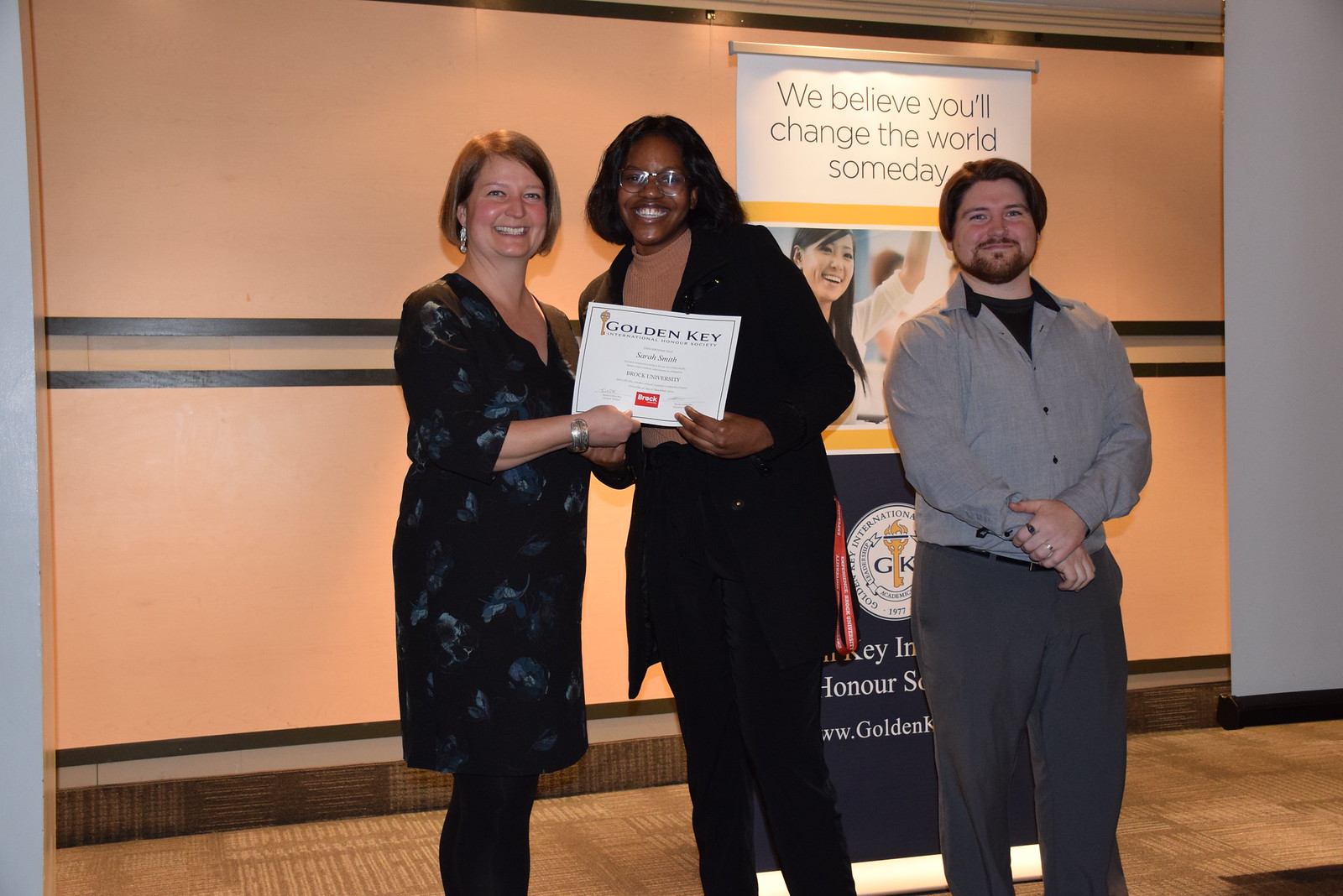This horizontal rectangular image captures a vibrant scene in an auditorium or meeting room with an orange wall featuring a stripe midway and a brown wood-tiled floor. Standing in front of a partially obscured sign that reads "We believe you'll change the world someday" at the top, are three individuals: two women on the left and a man on the right. The woman on the far left is a Caucasian wearing a dark blue dress that reaches her thighs, adorned with earrings and a big smile. She is handing a certificate that reads "Golden Key" to the woman in the middle, who is African-American, has glasses and black hair, and is also smiling. The man on the right, also Caucasian, sports a gray shirt, gray pants, a beard, and slightly long hair styled to the sides. His attire is complemented by a couple of rings, and he looks directly at the camera with a smile. The sign behind them, featuring a partially visible image of a woman with an upraised arm, along with the text, suggests a celebratory or honorific event, likely an award ceremony.